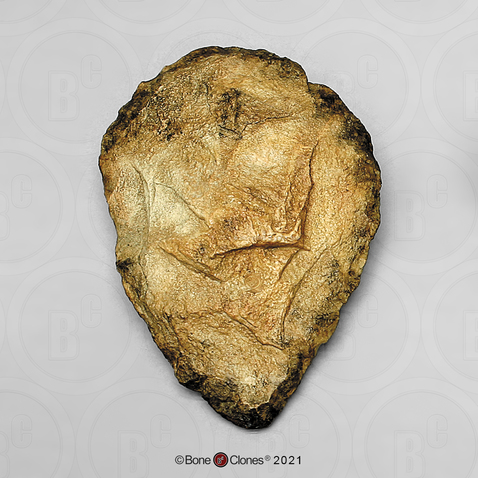The photograph features a close-up of an enigmatic artifact that closely resembles an arrowhead, but is more rounded, akin to a teardrop shape. The object, possibly a bone or a flake of rock, exhibits a dirty brownish-yellow hue with blackened edges that transition to a lighter interior. Prominently, the bottom of the artifact bears the text "© Bone Clones 2021," providing a clue to its origin or manufacturer. The setting of the image is a plain gray background, subtly interspersed with small "ABC" watermarks. The combination of these elements suggests an aged, possibly historical item, meticulously captured to highlight its texture and intricate details.